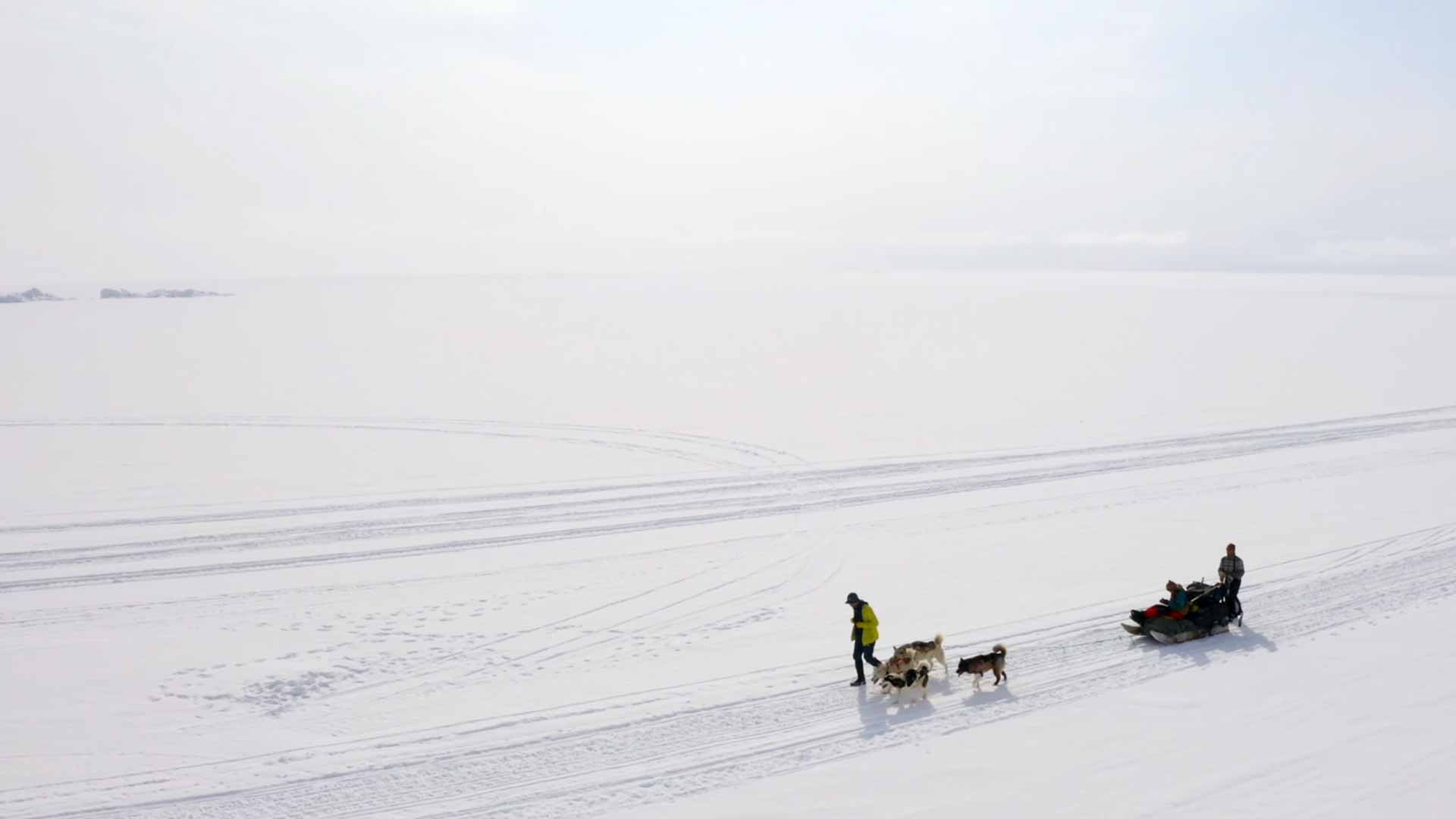The image captures a vast snow-covered tundra landscape, reminiscent of Alaska, with snow stretching as far as the eye can see, dominating approximately 75% of the scene. The remaining 25% is occupied by a bright, sun-bleached sky. Prominent in the foreground is a sled, pulled by four huskies, navigating through well-trodden tracks in the snow. Two people are involved: one in a yellow jacket walks alongside the dogs, while the other stands at the rear of the sled, steering it. There may also be a person seated within the sled, which is packed with supplies. The sled team is moving to the left of the frame, and their tracks blend seamlessly with other similar paths in the snow. The entire scene, devoid of any text or labels, evokes the harsh and beautiful isolation of arctic wilderness.